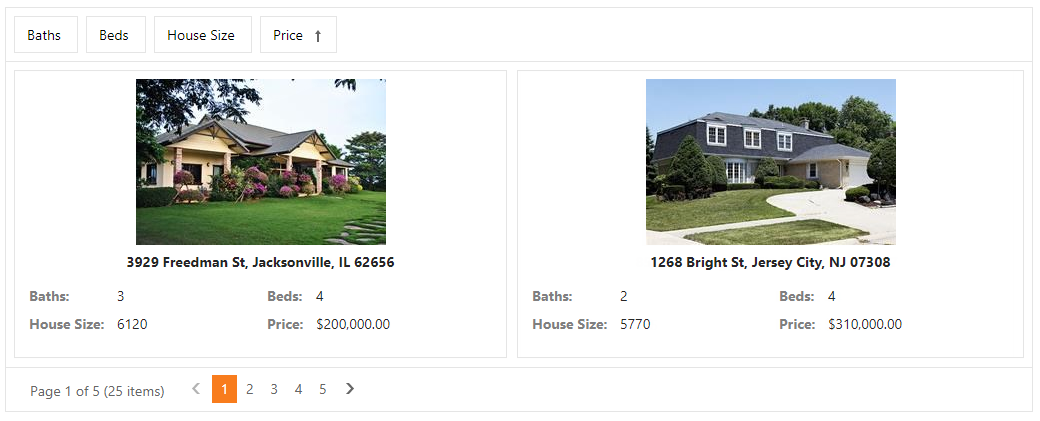This is a screenshot taken from a property comparison website, specifically from page 1 of 5, displaying a total of 25 listings. However, only 2 of these properties are visible in the screenshot. The first property listed is located at 3929 Freedman Street, Jacksonville, featuring 4 bedrooms, 3 bathrooms, and covering an area of 6,120 square meters, with a price of approximately $200,000. The second property is situated at 1268 Bright Street, Jersey City, NJ, boasting 4 bedrooms, 2 bathrooms, and a size of 5,770 square meters, priced around $310,000. 

At the top of the page, there are filtering options to sort search results by the number of bathrooms, bedrooms, house size, and price. The user is currently on the first page of their search, exploring available properties in diverse locations including Jacksonville and Jersey City.